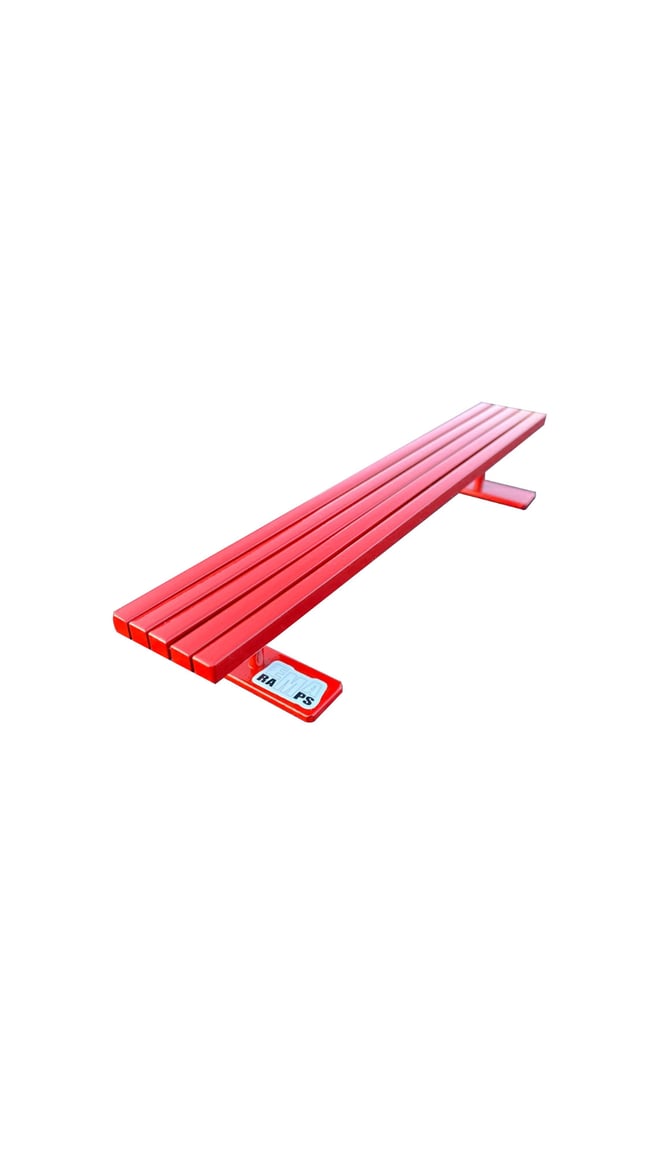The image showcases a red bench set against a solid white background. The bench is composed of five thin, rectangular strips made of either painted metal or wood, stacked horizontally with small gaps between each. This design is reminiscent of a park bench, though without a backrest. The bench is slanted, running from the bottom left corner to the top right corner of the image. Each end of the bench features short red rods that support the structure, connected to rectangular bases.

On the seat of the bench, there are markings: the letters "R.A.M.P.S." are visible, with "E.M.A." written in white over these black letters. The construction of the bench appears to give it a shiny finish, and it seems to fade into a lighter color towards the back, giving a sense of depth and elongation in the image.